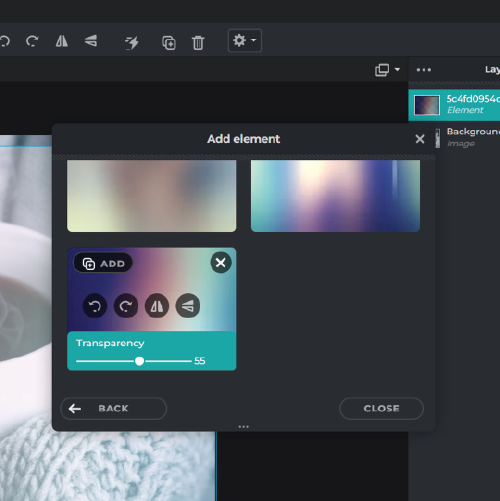The image showcases a close-up view of a screen with a predominantly black background and a vertical dark gray strip on the right side. In the background, one can discern a cropped photograph of a white coffee cup, partly filled with coffee, situated on the left side, partially cut off. Adjacent to the cup is a knitted white sweater, adding a cozy texture to the scene. 

Prominent in the center of the screen is an open dialog box displaying three images. The top two images are horizontally aligned and only partially visible, each featuring vibrant gradients of blue, purple, and pink hues. Below these, on the bottom left, is another image also characterized by a gradient background. This image is overlaid with a banner labeled "transparency" accompanied by a slider for adjustment.

Additionally, the dialog box contains several interactive elements. On the top left, there is an advertisement, with a small 'X' button for closing the ad in the top right corner. Across the middle of the box are four circular icons featuring different symbols. At the bottom, navigation buttons are present, with a back button on the left and a close button on the right.